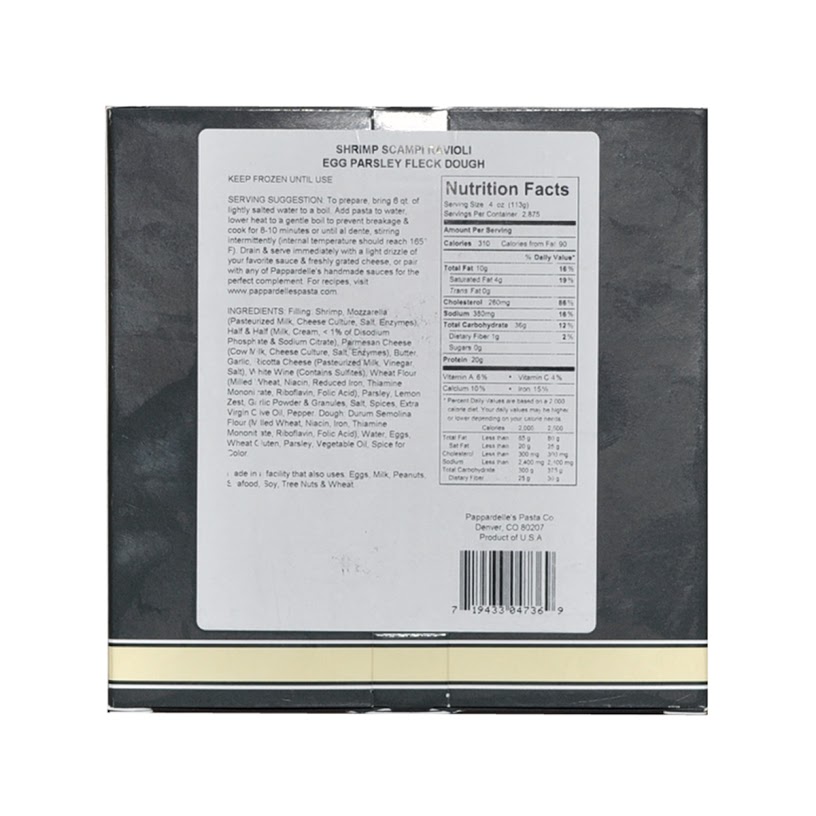This image captures the detailed label of a food package. The package itself is partially visible, with its top section being black and a cream-colored stripe running horizontally across the bottom. Prominently displayed on the package is a large white sticker containing essential product information. The label reads "Shrimp Scampi Ravioli" and mentions that the ravioli is made with egg and parsley-flecked dough. It advises to keep the product frozen until ready to use. 

For preparation, the label suggests bringing six quarts of lightly salted water to a boil, then adding the pasta, reducing the heat to a gentle boil to prevent breakage, and cooking for 6 to 10 minutes until al dente, while stirring occasionally. The internal temperature should reach 165°F. Once cooked, the ravioli should be drained and served immediately, with a light drizzle of your favorite sauce and freshly grated cheese. Alternatively, it can be paired with any of the handmade sauces recommended by the producer.

The bottom of the label indicates that the product is made by Pappardelle's Pasta Company, located in Denver, Colorado 80207, USA. The website and detailed nutrition facts are mentioned, but the tiny font makes them difficult to decipher.